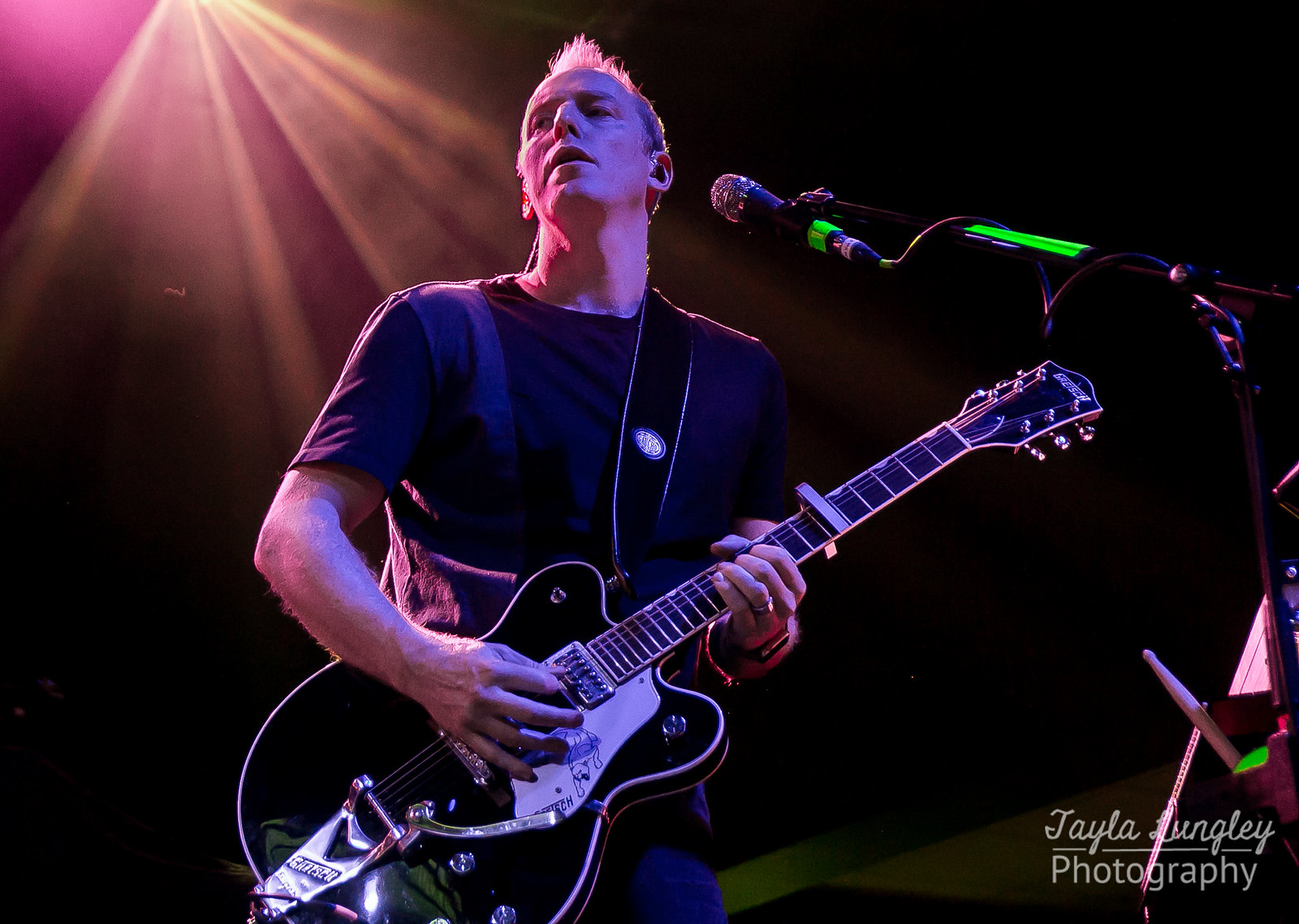The photograph captures a mid-concert moment of a middle-aged white guitarist performing on stage, immersed in shadows that render the background almost entirely black. A sharp beam of light from a ceiling-mounted spotlight illuminates the performer from the top left corner, creating a striking contrast. The musician, sporting short, spiky hair, is clad in a black short-sleeve crew neck t-shirt. A black strap secures a black-and-white electric guitar around his left shoulder, with one hand on the frets and the other strumming the strings. Positioned to the right, a black microphone stand, wrapped in green tape at various points, extends from the bottom right up to the center of the image, supporting a black microphone angled towards the guitarist’s face. Partially visible on the far right is the edge of a metal chair. The photograph is subtly signed with a see-through white watermark in the bottom right corner, reading "Taylor Lingley Photography" in cursive.